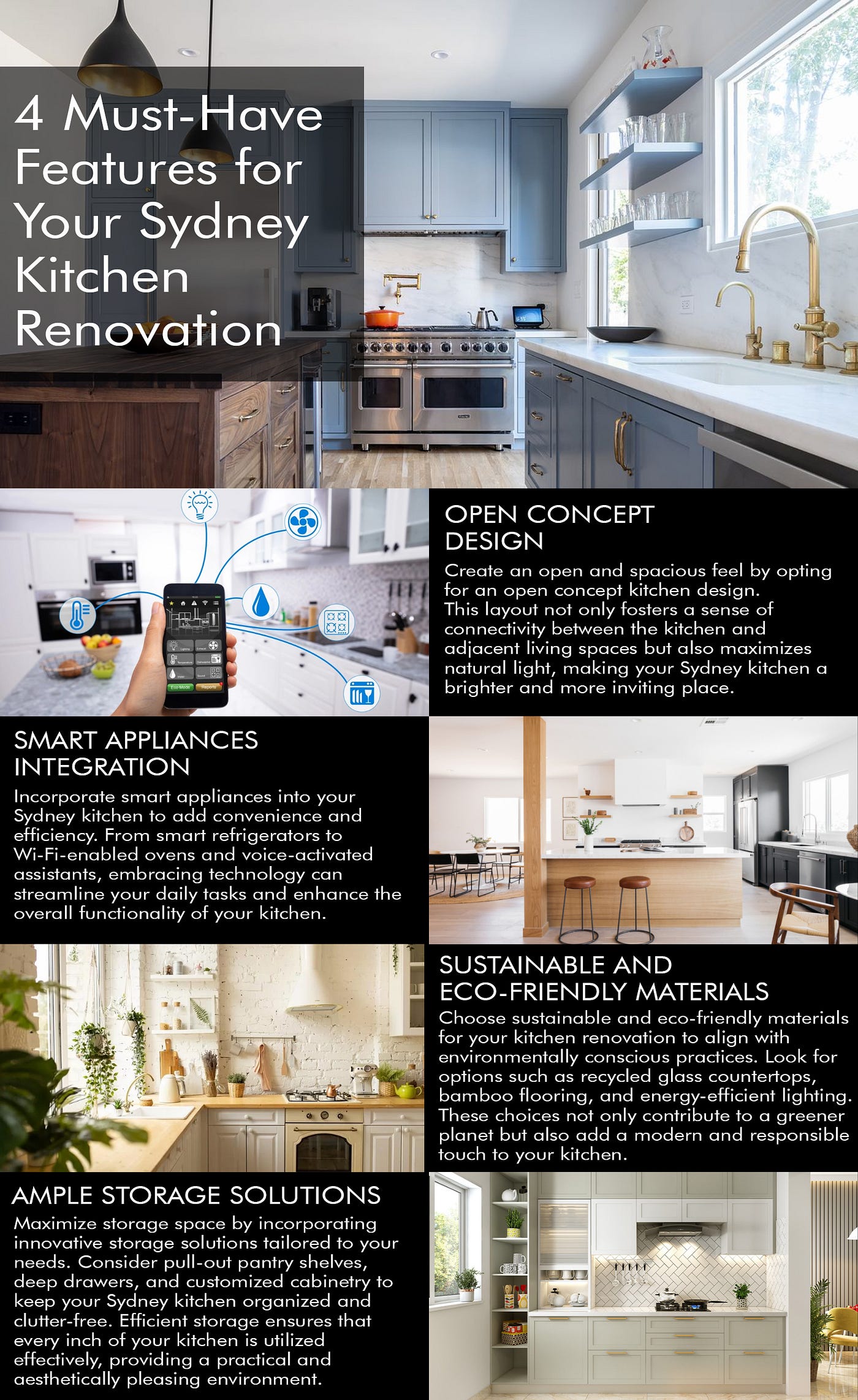This is a detailed photo advertisement for a kitchen renovation company in Sydney, Australia. The ad features five distinct, color photos of modern kitchens, each showcasing different key elements of an ideal kitchen remodel. The layout consists of vertical columns with each kitchen photo situated beside a black rectangle containing descriptive text in white font.

At the top of the advertisement, in large white lettering on a black background, it states: "Four Must-Have Features for Your Sydney Kitchen Renovation." Below, each kitchen photo is accompanied by text detailing a specific desirable feature:

1. **Open Concept Design**: The photo depicts a modern kitchen with an iPhone connected to various kitchen features. The text emphasizes creating an open and spacious feel, fostering connectivity between the kitchen and adjacent living spaces, and maximizing natural light to make your kitchen brighter and more inviting.

2. **Smart Appliances Integration**: This image shows a modern kitchen with an island. The text highlights the convenience and efficiency of incorporating smart appliances, such as smart refrigerators, Wi-Fi enabled ovens, and voice-activated assistants, to streamline daily tasks and enhance kitchen functionality.

3. **Sustainable and Eco-Friendly Materials**: The photo illustrates another contemporary kitchen design, focusing on eco-conscious choices. The accompanying text suggests using recycled glass countertops, bamboo flooring, and energy-efficient lighting, contributing to a greener planet while adding a modern and responsible touch to the kitchen.

4. **Ample Storage Solutions**: The final image showcases an interior kitchen view with innovative storage options. The text recommends maximizing storage space with pull-out pantry shelves, deep drawers, and customized cabinetry to keep the kitchen organized and clutter-free, ensuring every inch of space is utilized effectively for a practical and aesthetically pleasing environment. 

Throughout, the advertisement presents bright, sunny kitchens featuring modern cabinets and appliances, designed to inspire and guide homeowners in their Sydney kitchen renovation projects.